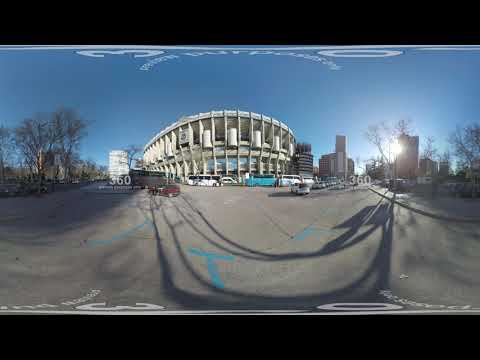The image captures a distorted 360-degree panoramic view of an urban setting on a sunny day. Central to the image is a large, rounded building that resembles either a stadium or a convention center. The curved fisheye lens skews the perspective, making one side of the building appear significantly larger than the other.

Surrounding the main structure is a gray pavement parking lot with a few parked cars and visible shadows of leafless trees. The trees are positioned on both the left and right sides of the image, with some taller buildings rising in the background. Among these structures, the sun is prominently visible on the center-right, casting strong light and creating dramatic shadows on the pavement below.

In the foreground, numerous cars and buses, each with distinctive colors such as red and white, are seen moving along a street that runs in front of the central building. The fisheye effect causes the shadows and the text on the pavement – featuring letters like a capital 'T' and numerals such as a sideways '3' and '0' – to appear curved and distorted, stretching across the image in a U shape. Additionally, there are black borders on both the top and bottom of the image, emphasizing the panoramic aspect of the scene.

Overall, this 360-degree photo provides a comprehensive, albeit skewed, view of a bustling area featuring a prominent stadium-like building, a busy street with vehicles, and a mix of barren trees and tall buildings framed against a clear, blue sky.